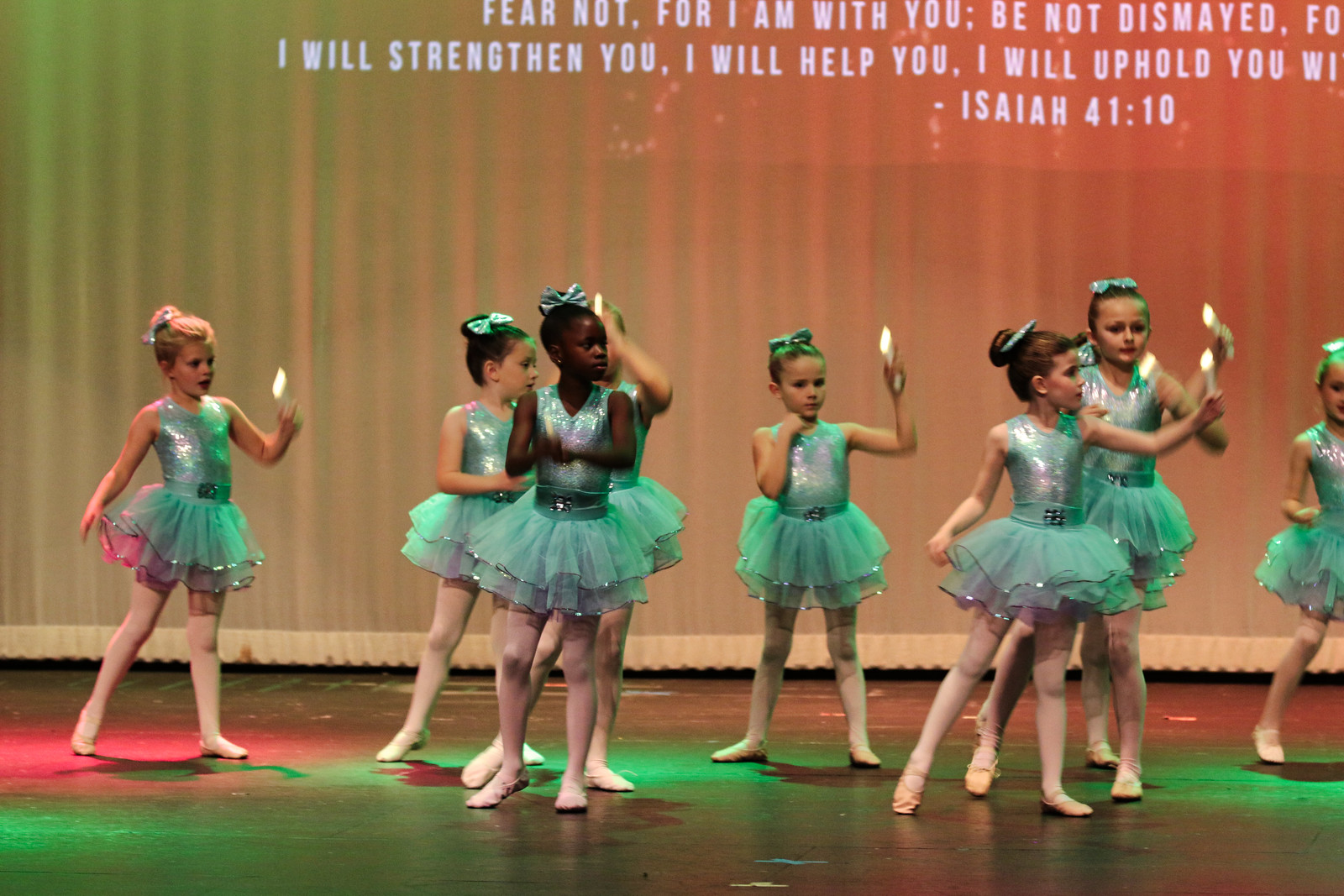The image captures a lively stage performance featuring several young girls, approximately 10 years old, dressed as ballerinas. They are adorned in shiny emerald or sea-green tutu dresses with lacy, frilly skirts and gold-trimmed edges. Each girl has ribbons in their braided hair and wears ballerina shoes. They perform under a mix of red and green lights that illuminate the stage, casting colorful hues on their outfits. Some girls are holding objects that emit light, though these appear blurred due to movement. A partially visible biblical quote from Isaiah 41:10 is projected on the curtain behind them, reading, "Fear not, for I am with you; be not dismayed, for I will strengthen you, I will help you, I will uphold you."